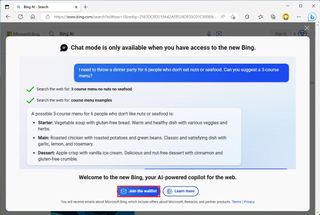At the top of the image, there is a gray area which is small and blurry, making it difficult to decipher any text within it. Along the tab at the top, some text is visible, and a URL is present in the address bar. Additionally, several icons are displayed in the browser's top section. The image shows a web browser displaying a pop-up window with a message stating, "Chat mode is only available when you have access to the new Bing," accompanied by a black checkbox next to this statement. Below the checkbox is a long, rectangular blue box containing some text, but it is too blurred to read clearly. Further down, there are two lines, each with a green checkmark beside them, though the text is also indistinct. Beneath these elements is a box with a line at the top, followed by three bullet points, each accompanied by a short sentence. At the bottom of this section is a standalone sentence, followed by two buttons—one blue and one white.